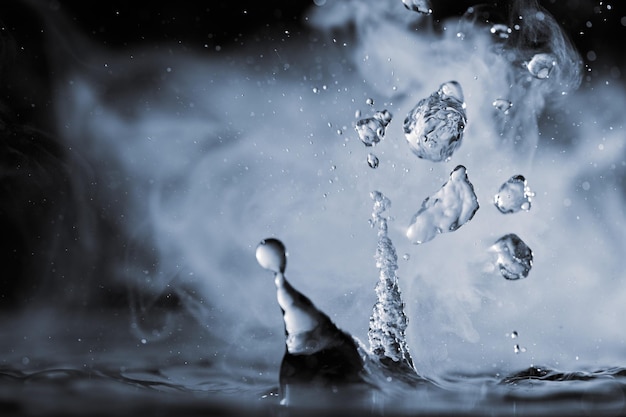This detailed, close-up color photograph captures the dramatic moment of a water splash set against a completely black background. A swirling, white mist or haze adds an almost menacing fog-like atmosphere behind the action. In the foreground, multiple droplets can be seen in mid-motion, suspended above the water surface. The centerpiece is a large splash with a prominent droplet perched at the top, while a smaller, cone-shaped splash with drops protruding upward is situated beside it. To the right, two medium-sized globs of water anchor the composition, with additional droplets radiating outward in various sizes and directions, as if the water were struck forcefully and sent bursting into the air. The chaotic beauty of the water droplets and the play between the dark background and white mist create an abstract, yet vividly dynamic scene.